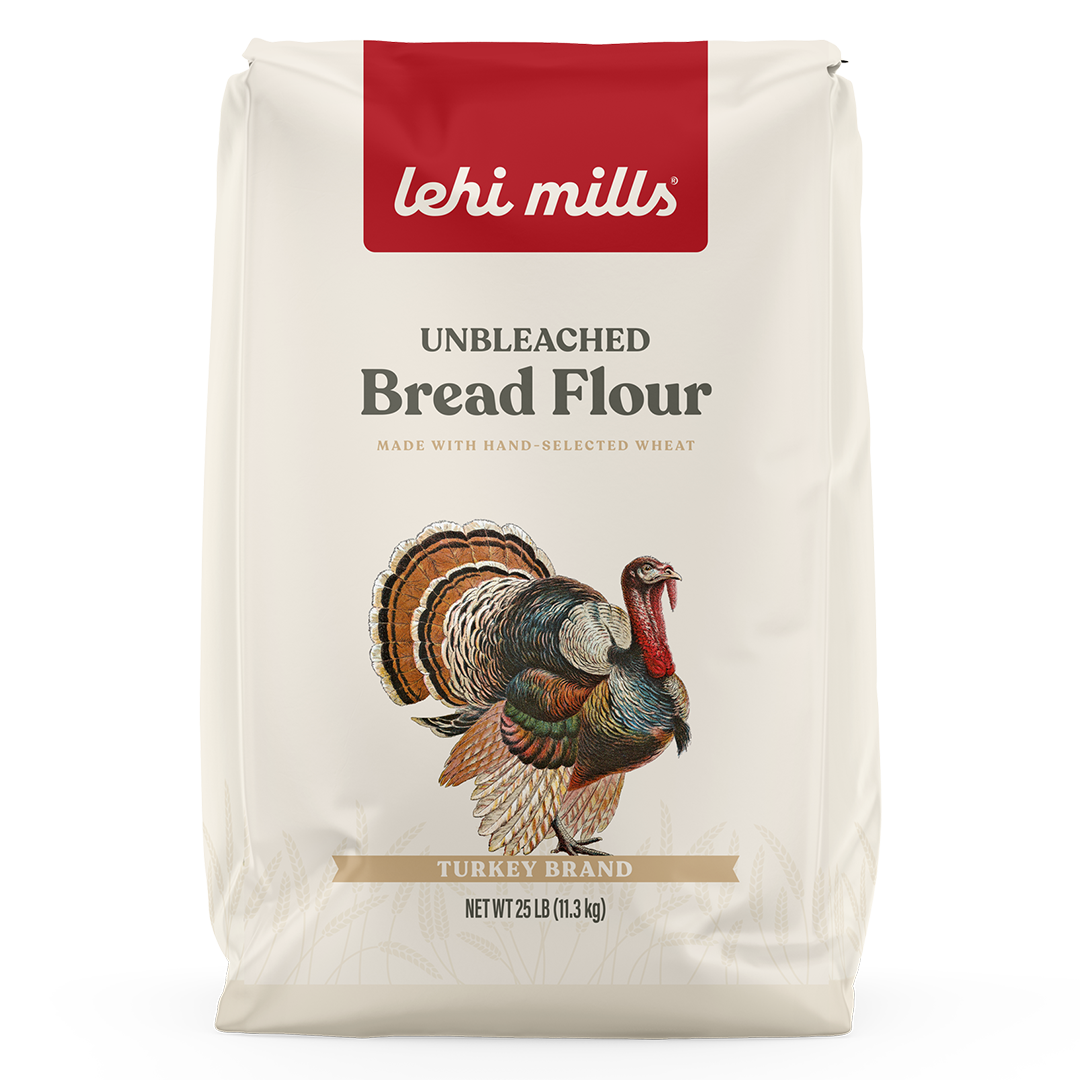The image depicts a large, rectangular, white paper bag of Lehigh Mills Unbleached Bread Flour. The top of the packaging prominently features the Lehigh Mills logo, which is a big red rectangle with white lettering. Below this, in dark gray and tan tones, the text reads "Unbleached Bread Flour" and "made with hand-selected wheat." Central to the design is a colorful, drawn image of a male turkey, characterized by a vibrant red neck and multicolored feathers, facing towards the right. Underneath this illustration, the text "Turkey Brand" is visible. The bottom of the bag specifies the weight of the flour as "Net Weight 25 lbs (11.3 kg)" in black font. The entire design is set against a simple, white background, making the detailed and colorful depiction of the turkey stand out.